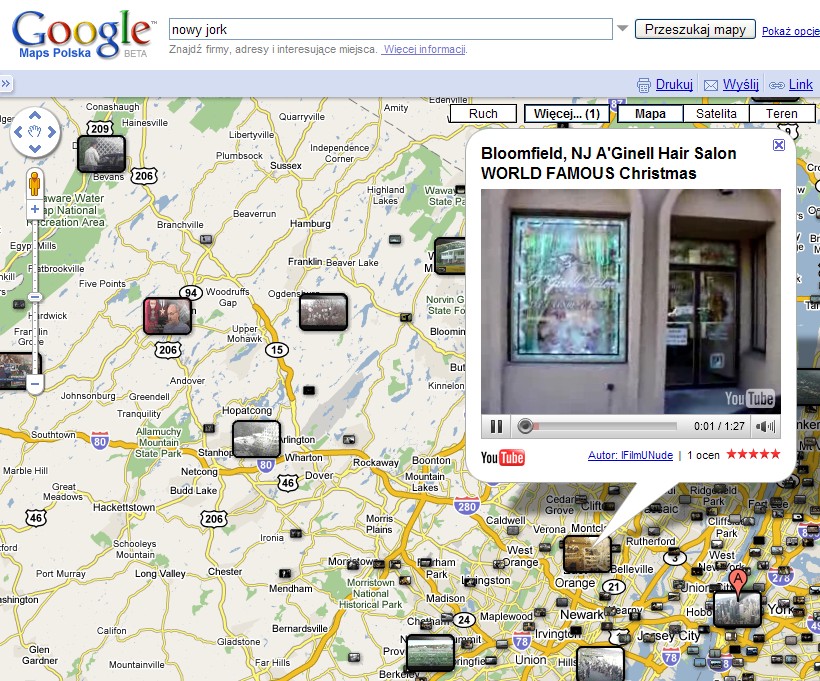Google Maps Polska interface showing a search result for "Nowy York." The primary image consists of a detailed map with roads highlighted in yellow against a white background, characteristic of standard map designs. A series of rectangular images overlays the map, presumably representing various locations. On the right side of the image, there is a prominent white pop-up box displaying search results. Notably, this box lists "Bloomfield, New Jersey," followed by specific points of interest such as "Janelle Hair Salon" and "World Famous Christmas." The pop-up features a square image resembling a YouTube video, complete with a YouTube logo, gray progress bar, and five red stars in the bottom right corner, signifying ratings. Additionally, several black squares, scattered throughout the map, seem to mark key locations, including one with a red teardrop icon marked with the letter 'A.' The entire scene resembles an older version of a Google Maps results page.